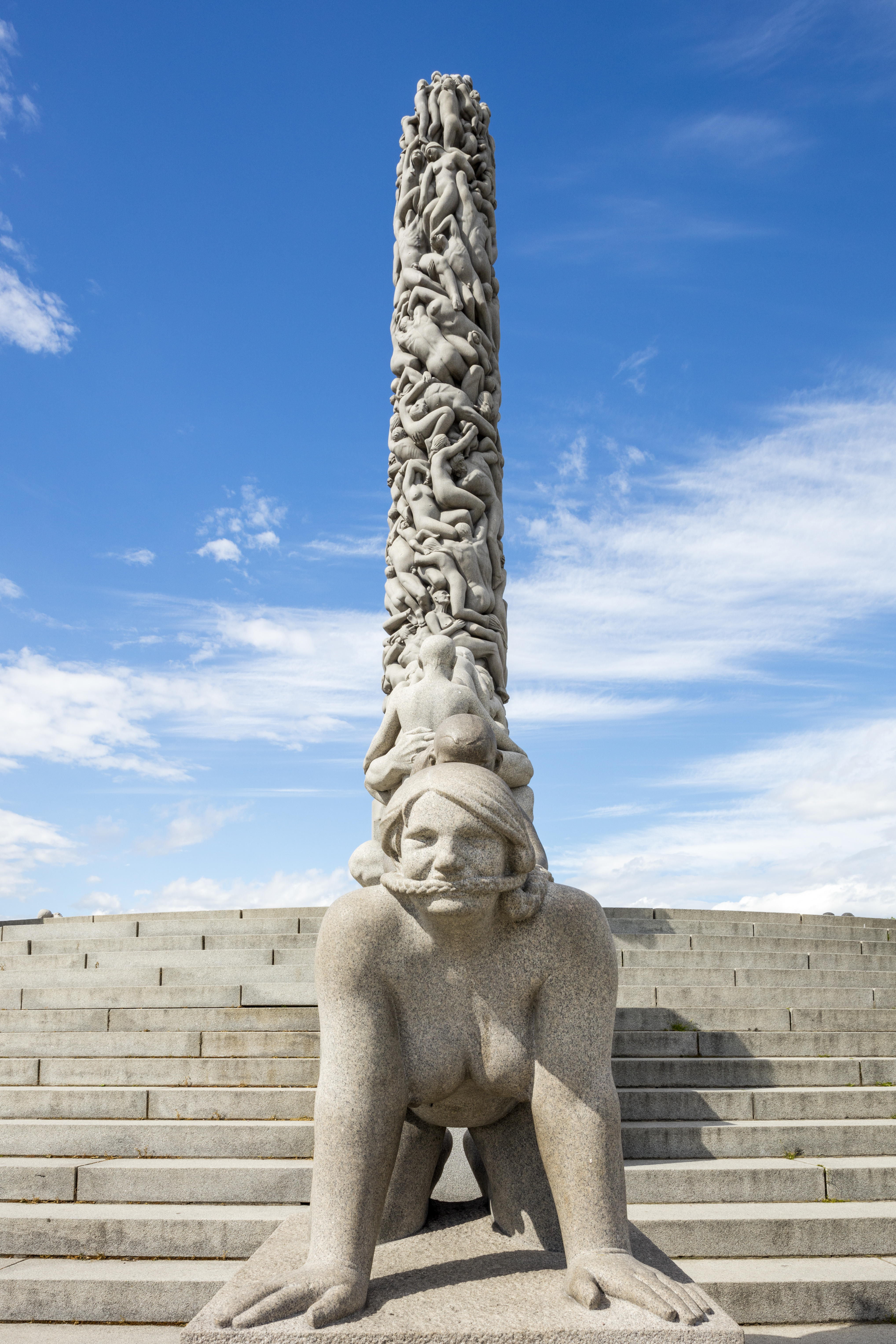The image features a large and intricate sculpture situated outdoors, displayed against a backdrop of blue sky punctuated by a few white clouds. The sculpture is positioned in front of a set of substantial gray stone steps. At the base of the steps, there is a flat platform where a female figure is depicted on her hands and knees, facing forward. The female figure has shoulder-length hair and is crafted from the same gray stone as the steps. Emerging from the top of her head is a cylindrical tower composed entirely of intricately interwoven stone bodies, tightly packed together to form a cohesive tube-like structure. Additionally, a chain or rope is depicted stretching across the woman's mouth, extending back on each side of her face. The craftsmanship of the statue is highly detailed, with the stone bodies that make up the tower showing meticulous sculptural work.